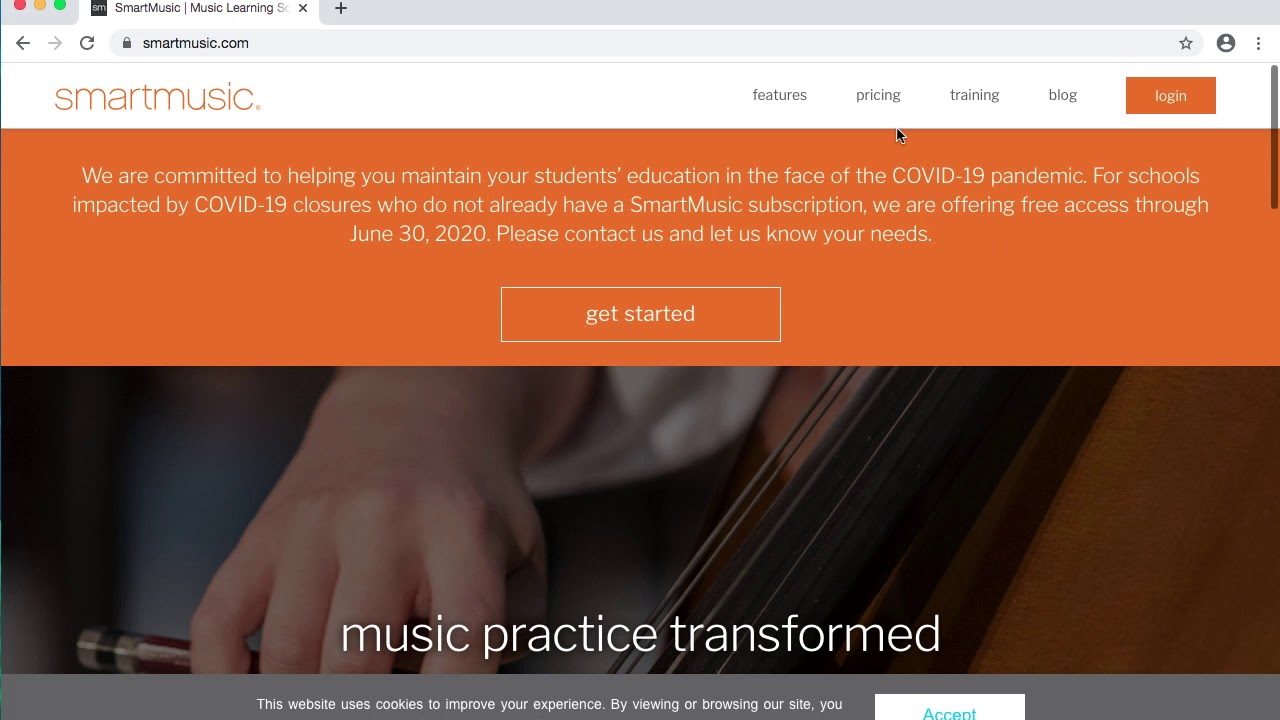Screenshot of a Macintosh computer displaying the Smart Music website. In the top-left corner, familiar red, orange, and green circles confirm the Mac interface. On the right side, a dark gray bezel features a tab labeled "SM" in white text on a black square, followed by "Smart Music," a vertical line, "Music Listening," and a cut-off "S." An "X" icon is also visible. Below, in a white bezel, a black back arrow and a gray forward arrow indicate navigation buttons alongside a refresh arrow loop. The mid-gray URL bar shows a secure black lock symbol next to "smartmusic.com." At the far right, a star bookmark icon, a profile circle, and three ellipses for settings are presented.

In the main content area, a white rectangle with "Smart Music" and an orange dot is visible on the left. To the right, tabs with black text read "Features," "Pricing," "Training," "Log," and the last one in orange with "Log In." Below, an orange banner with white text states, "We are committed to helping you maintain your student's education in the face of the COVID-19 pandemic. For schools impacted by COVID-19 closures who do not already have a Smart Music subscription, we are offering free access through June 30th, 2020. Please contact us to let us know your needs." A central button invites users to "Get Started" in bold white text. 

A light-skinned hand wearing a white undershirt and blue pants is partially visible, overlaid with the text "Music Practice Transformed." A dark gray section below reads, "This website uses cookies to improve your experience by viewing and browsing our site you," which is cut off. Finally, a white rectangle with cyan blue accents and partial text concludes the visible information.